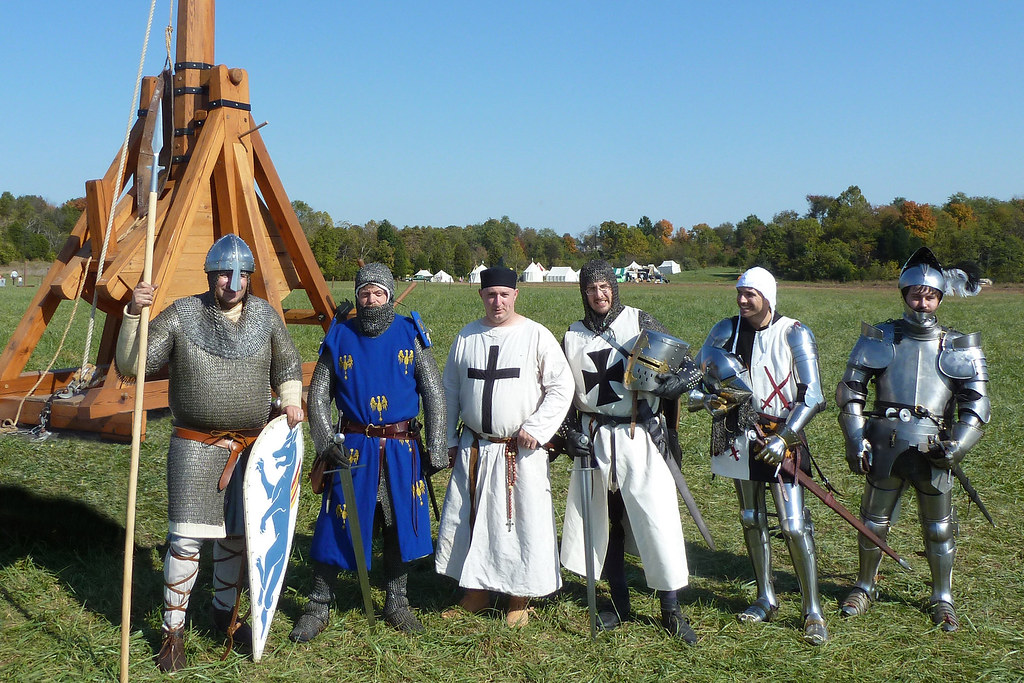This photograph captures six men engaging in medieval roleplay, dressed in detailed medieval garb, standing in a lush green field that occupies the lower two-thirds of the frame. On the left side is the base of a reddish-brown wooden trebuchet. From left to right, the first man is clad in a knee-length chain mail shirt, gray pants with brown straps, and a silver helmet with a large nose guard. He holds a light beige spear with a silver tip in his right hand and a white kite shield adorned with a blue horse, pinned to the ground with his left hand. Next to him is a man wearing a blue overcoat over a chain mail shirt, with chain mail boots and a hood. He holds a silver sword pointed toward the ground in his right hand. The third man wears a white cassock with a prominent black cross on the front and a black cap, topped off with beige shoes. Beside him stands another man in a chain mail shirt and hood, with a white overcoat featuring a black square cross with flared edges. He holds a silver helmet with a gold cross in his left arm and a simple sword pointed to the ground in his right hand. To his right, a man is outfitted in plate armor beneath a checkered shirt of black and white squares, holding a pointed-nose helmet in his right hand and the hilt of a sword and a leather scabbard in his left. The final man is in full plate armor, without any overlying cloth. All men are smiling at the camera, with a medieval wooden structure reminiscent of a trebuchet visible in the background, and trees and grass surrounding them.